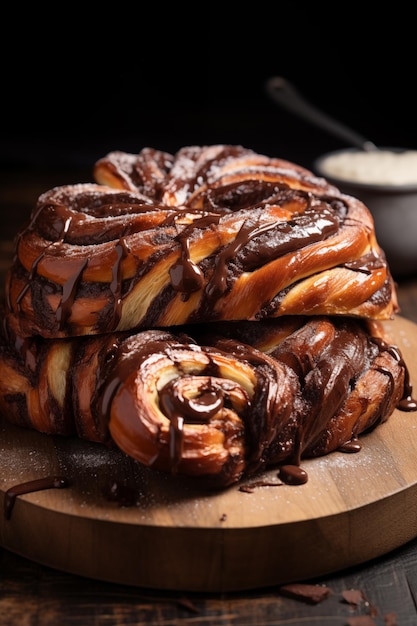This photographic, indoor setting captures a mouth-watering cinnamon roll that could easily be mistaken for a Cinnabon delight. The dense, golden-brown pastry showcases a glossy sheen, courtesy of a sugar glaze that reflects the camera flash. The cinnamon roll's layers are intricately coiled, with one part slightly open, revealing its textured, cinnamony interior. Dark streaks of rich chocolate adorn the roll, adding a decadent touch.

The roll is perched on a circular wooden cutting board, which features darker brown bands and provides a rustic charm. This cutting board rests on a well-used brown wooden table that has a mix of lighter and darker tones, likely worn and scratched over time. Scattered crumbs hint at the deliciousness of the treat above.

In the background, there's a slightly blurred bowl containing a white substance, possibly sugar cubes or oatmeal, set against a black backdrop that accentuates the vibrant details of the foreground. The entire image is text-free, focusing all attention on the luscious dessert and its inviting setting.